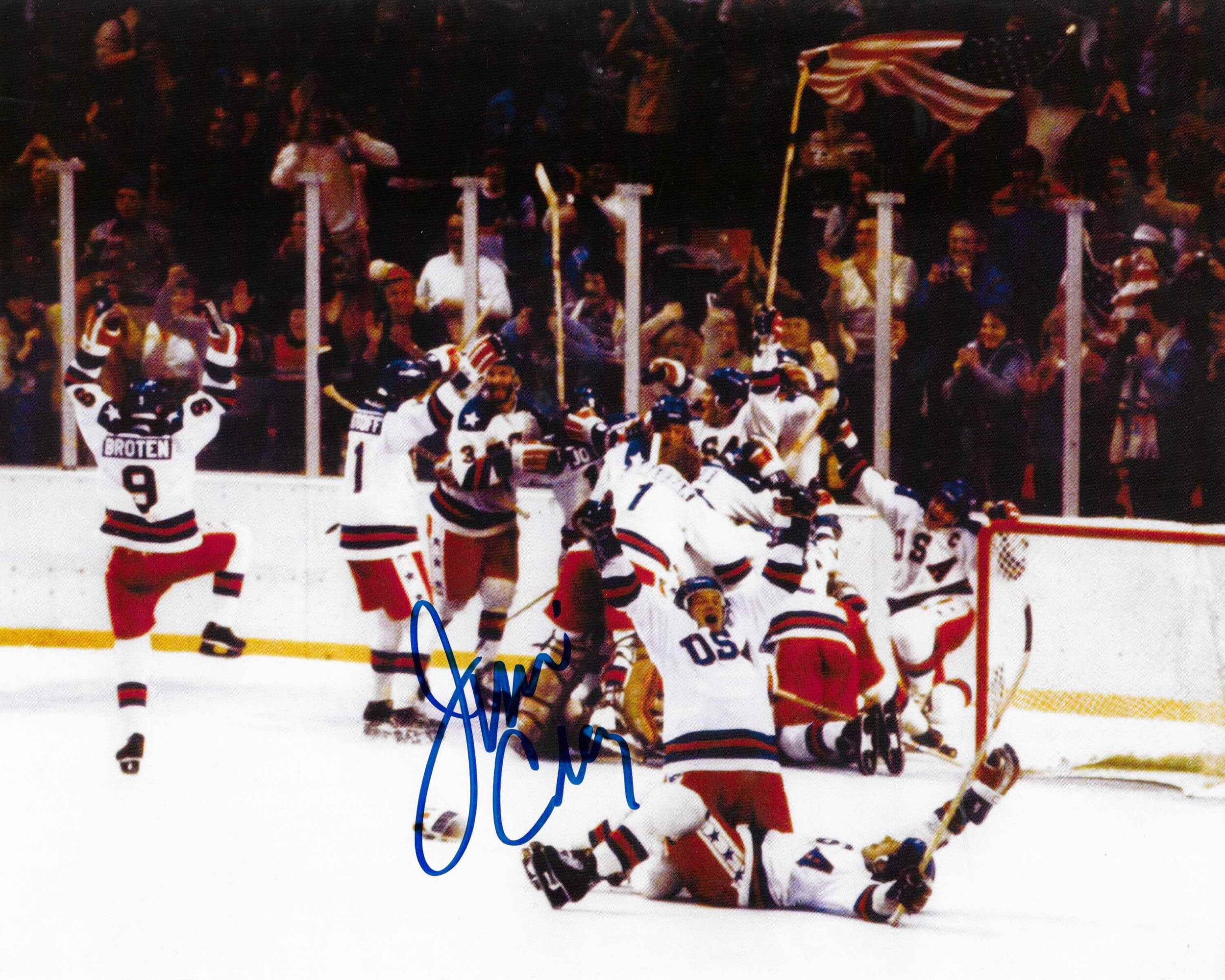The photograph captures the exhilarating moment of the 1980 "Miracle on Ice," where the United States hockey team triumphed over the Soviet Union. The victorious players, wearing white jerseys adorned with "USA" and red shorts over black leggings, are seen in various exuberant poses—jumping, hugging, and lying on the ice. One notable player, with the number 9 and the name "Broten" on his back, is celebrating with one foot in the air and arms raised. The background is filled with jubilant spectators standing behind the plexiglass, one proudly waving an American flag. The image features a prominent blue ink autograph, likely from Jim Craig, the renowned goalie of the team. The celebratory frenzy captures the essence of this historic win, with sticks held high and pure joy etched on the face of every player.